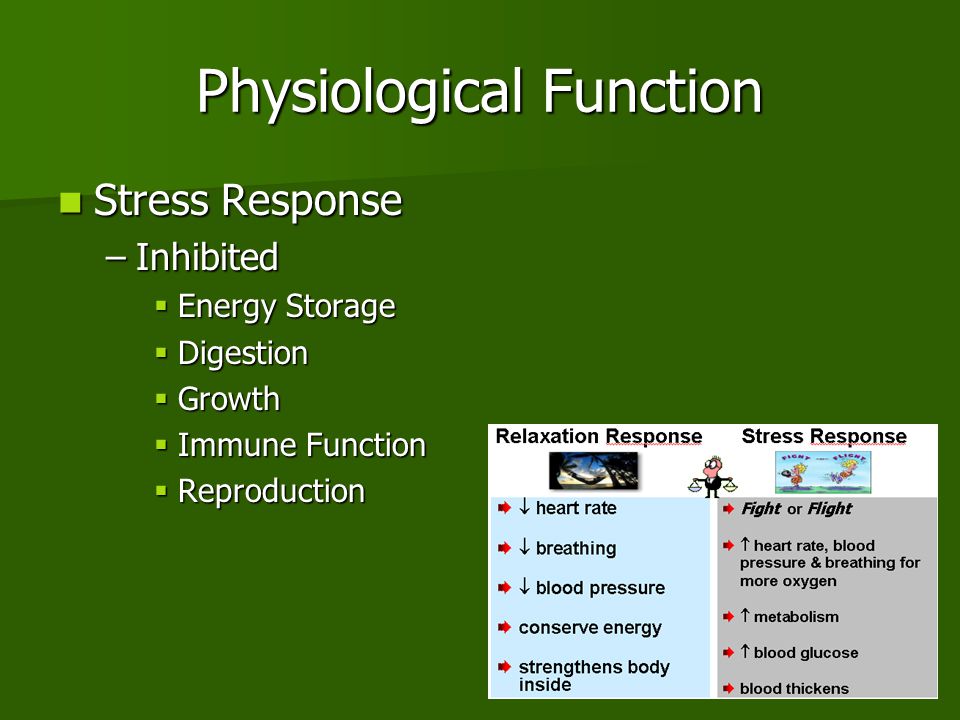The PowerPoint slide features a hunter green background with white text. At the top, the title reads "Physiological Function." Underneath, it highlights "Stress Response" followed by "Inhibited," and then lists key physiological processes: "Energy Storage," "Digestion," "Growth," "Immune Function," and "Reproduction."

In the bottom right corner, there is a square with a subdivided white, blue, and gray background. On the left side, under the header "Relaxation Response," the text lists "Heart Rate" with a down arrow, "Breathing" with a down arrow, "Blood Pressure" with a down arrow, "Conserve Energy" (no arrow), and "Strengthens Body Inside." 

On the right side of the square, under the header "Stress Response," it details the "Fight or Flight" mechanism, indicating increases with up arrows in "Heart Rate," "Blood Pressure," "Breathing for More Oxygen," "Metabolism," and "Blood Glucose," alongside the note "Blood Thickens" (no arrow).